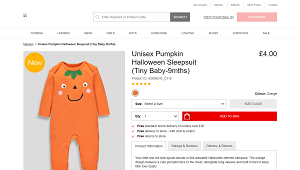This image features a blurry webpage showcasing a Halloween-themed baby costume. Dominating the left side of the page is a picture of a small, bright orange jumpsuit designed to resemble a pumpkin. The costume includes charming details such as green leaf accents on the front and a jack-o'-lantern face complete with two eyes, a nose, and a smiling mouth. The descriptive text for the item reads: "Unisex Pumpkin Halloween Sleep Suit for Tiny Baby," and it is marked as a new product. The price of the jumpsuit is displayed to the right, which is $4. Below this price, there are various dropdown buttons, likely for selecting size or quantity. Additionally, there is a prominent red "Add to Bag" button, indicating it is a clickable option for purchasing the item. The surrounding text on the webpage remains indistinct due to the blurriness.